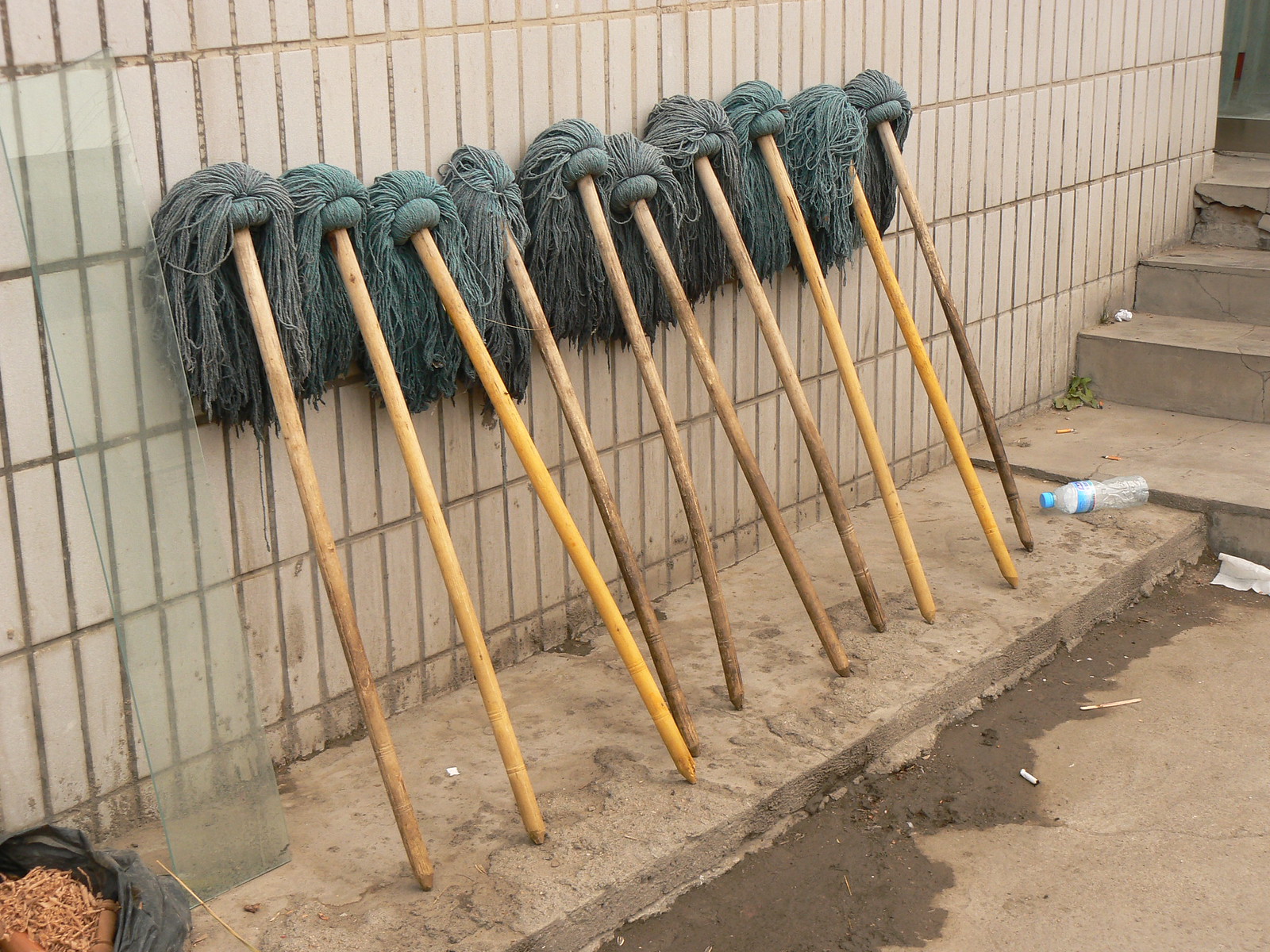In this photo, we see a row of 10 weathered mops leaning up against a light tan tile wall, composed of long, skinny rectangular tiles meticulously laid in rows. The wall is increasingly dirty at the bottom, marred with splatters of brown dirt. The mops feature long wooden handles, varying in shades from light brown to light yellow, some appearing more dirt-streaked than others. The mop heads are gray, resembling tangled strands of hair or dreadlocks, adding to the overall grungy aesthetic. The mops rest on a narrow, dirty sidewalk, speckled with cigarette butts and debris, including a discarded plastic bottle to the right of the mops. Further to the right, a stone staircase with visible cracks ascends to a green door, and nearby, a large pane of glass leans against the wall. The scene extends to a small parking lot area, littered with muddy water and trash, evoking a sense of neglect and utilitarian decay.